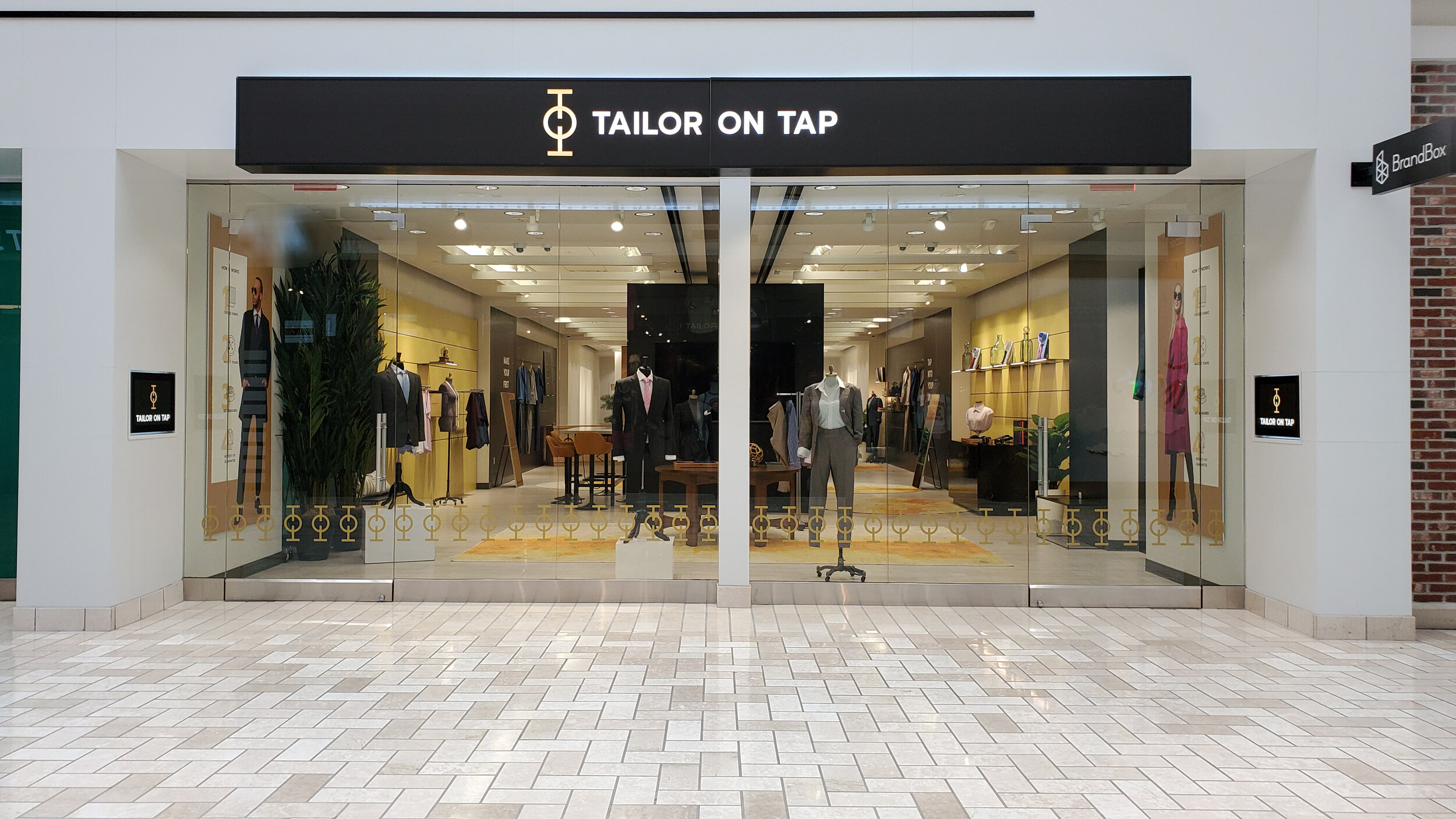The photo captures the storefront of "Taylor on Tap," presumably located within an indoor mall, given its pristine white tile flooring and clean, sharp white walls. The store's entire frontage is floor-to-ceiling glass, providing a full view of its well-lit interior. The store's name, "Taylor on Tap," is prominently displayed in white letters on a dark rectangular header above the entrance. The entrance features glass doors on either side. Inside, the store showcases a minimalistic and organized layout, with a focus on men's fashion. Two headless mannequins are prominently displayed at the front, dressed in a black suit and a gray suit, respectively. Along the walls are additional suits and jackets, hung neatly on hangers. The interior is brightly illuminated with lights from the ceiling, creating a vibrant and inviting atmosphere. To the right of the store, there is an additional sign reading "brand bar," fixed horizontally against the wall.